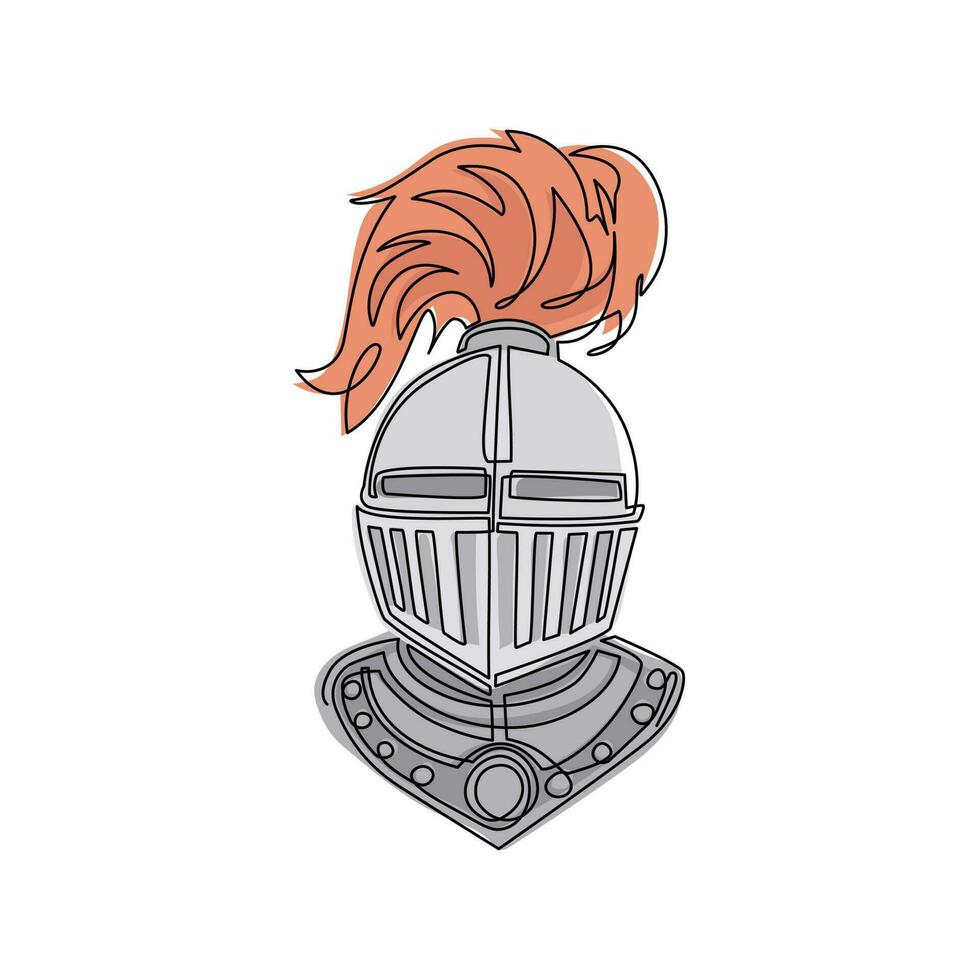This illustration showcases a detailed knight's helmet centered against a white background. The helmet features a striking burnt orange plume emerging from the top, outlined in black, giving the appearance of flames or feathers. The face of the helmet is designed with narrow, vertical slits for the eyes, providing a menacing and resolute look. The helmet itself is predominantly silver with varying shades of gray—the face area in a lighter gray and the neck and shoulder portions in a darker gray. Each segment is meticulously outlined in black details. The neck guard, which extends down to a pointed angle, is adorned with small decorative dots. The illustration, which might be hand-drawn or computer generated, includes subtle, intricate touches such as circles on the front and sides of the neck area, providing an additional layer of ornamental craftsmanship.